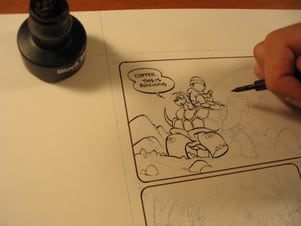In this detailed image, we observe a person meticulously drawing a comic strip on white paper that rests on a brown wooden surface. The scene captures the artist's steady hand holding a marker or pen in the upper right corner, as they outline and darken elements within the cartoon panels. 

The comic strip features two distinct rectangular panels, with the left side of the first panel already inked and the right side still showing pencil sketches. The depicted scene includes a man, a boy, and a dog riding on the back of a turtle, which appears to be moving to the right. Above them, in the first panel, there’s a text bubble that reads, “coffee this is,” followed by an unclear word starting with an “R.”

In the top left-hand corner of the paper, sits a black inkwell or bottle of ink with a tapered neck and white writing on it, which isn't fully legible. The overall setting and the partially inked drawings emphasize the process of bringing a cartoon to life, highlighting the intersection of creative preparation and detailed execution.